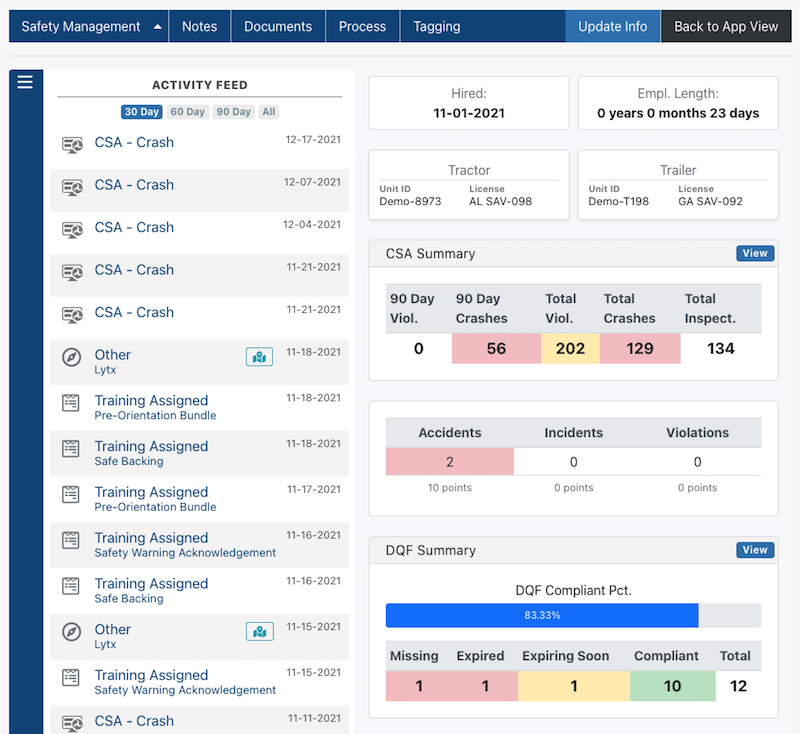In this image, we can see a detailed screenshot of an activity-oriented website interface. At the top right corner, there's a button labeled "Back to App View" in white text on a black background, beside another button labeled "Update Info" in white text on a light blue background. To the left of these buttons are menu headers for "Tagging," "Process," "Documents," "Notes," and "Safety Management," all displayed in white text.

On the middle left vertical section, there are several subsections labeled "CSA Crash," each with accompanying dates. The first entry states "CSA Crash" with the date "12-17-2021" on the right. Following rows repeat the "CSA Crash" label until the fifth entry, which then changes to "Other" with the date "11-18-2021."

In the top right section, there are four distinct rectangular areas. The first rectangle shows "Hired 11-1-2021." The rectangle directly to the right provides the "Employee Length," specified as "0 years, 0 months, 23 days." The bottom-left rectangle is labeled "Tractor," while the bottom-right rectangle is labeled "Trailer." Beneath these, there is a section titled "CSA Summary."